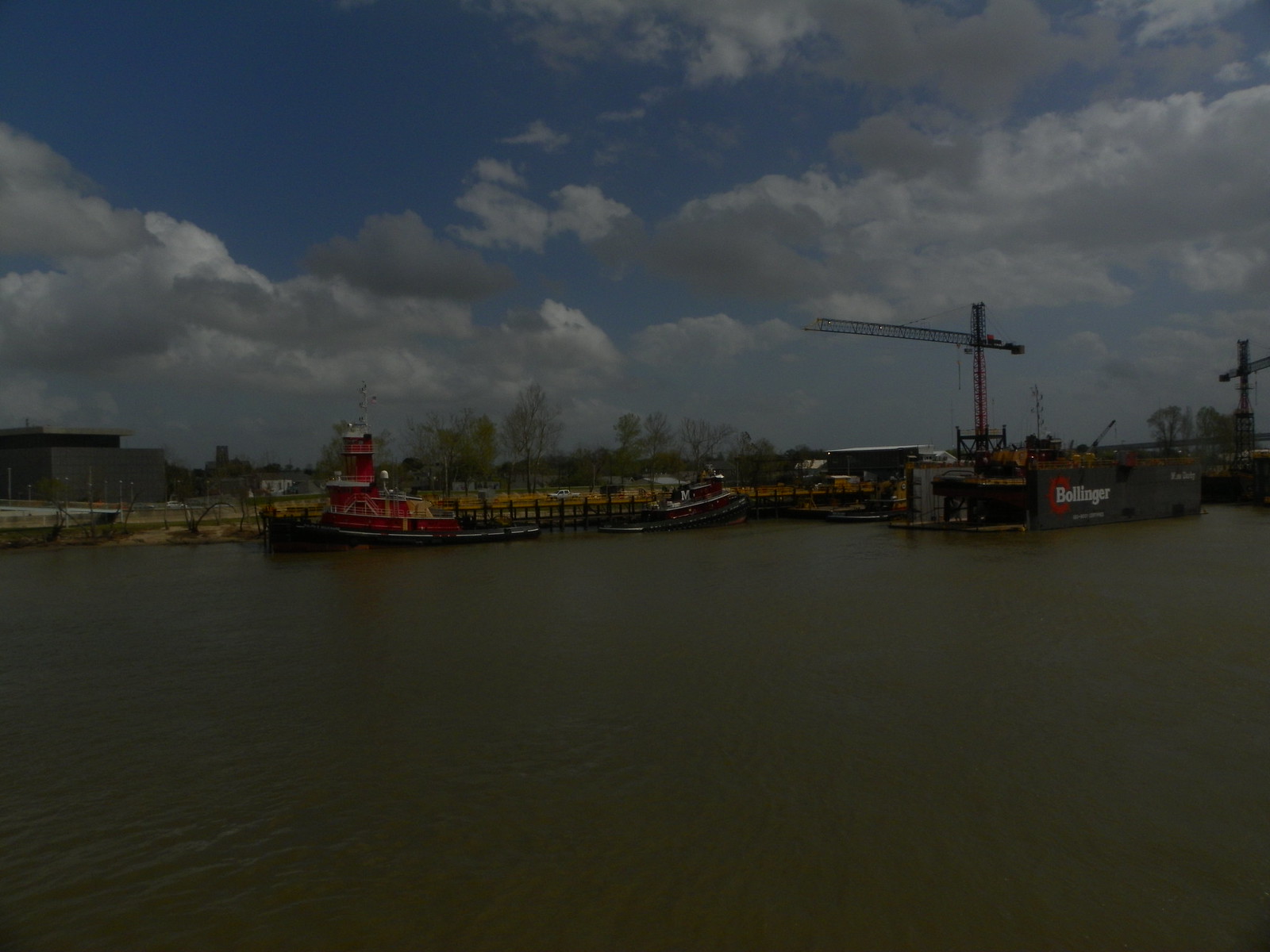This outdoor image features a vast sky filled with a mix of bright white and gray clouds above a dark, murky expanse of green-brown water. Dominating the mid-ground is a bustling pier or dock area, where two tugboats, painted in shades of red and maroon, are moored. They appear to be close to a bright yellow and black structure. Prominently displayed within the water is a sign for the company Bollinger, written in white text. In the background, a diverse skyline of buildings varies in height, interspersed with scattered trees, some bare and others covered in leaves. Adding to the industrial feel, two construction cranes rise into the sky, one with a red base transitioning to black. The scene is completed by the sight of a few cars traversing a nearby street.